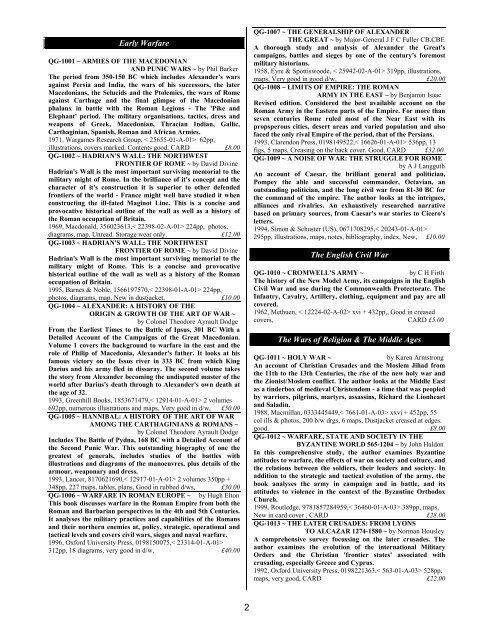This black and white image, resembling a page from a catalog or reference book, features small, densely packed text arranged in two columns. At the top left, under a black border, it reads "Early Warfare" and lists multiple sections, starting with "QG1001, Armies of the Macedonian and Punic War, by Phil Barker," followed by "QG1002, Hadrian's Wall, the Northwest Frontier of Rome, by David Divine," and several more, totaling six sections on this side. On the right column are seven additional sections. The content covers various historical warfare periods, including detailed headings like "Early Warfare," "The English Civil War," and "Wars of Religion and the Middle Ages," each accompanied by a few listings that likely describe books or texts, potentially available for purchase, indicated by prices in pounds. The bottom of the page indicates it's "Page 2" from a larger text, possibly a catalog or book on early warfare, with three main headers giving a structured overview of the historical content offered.